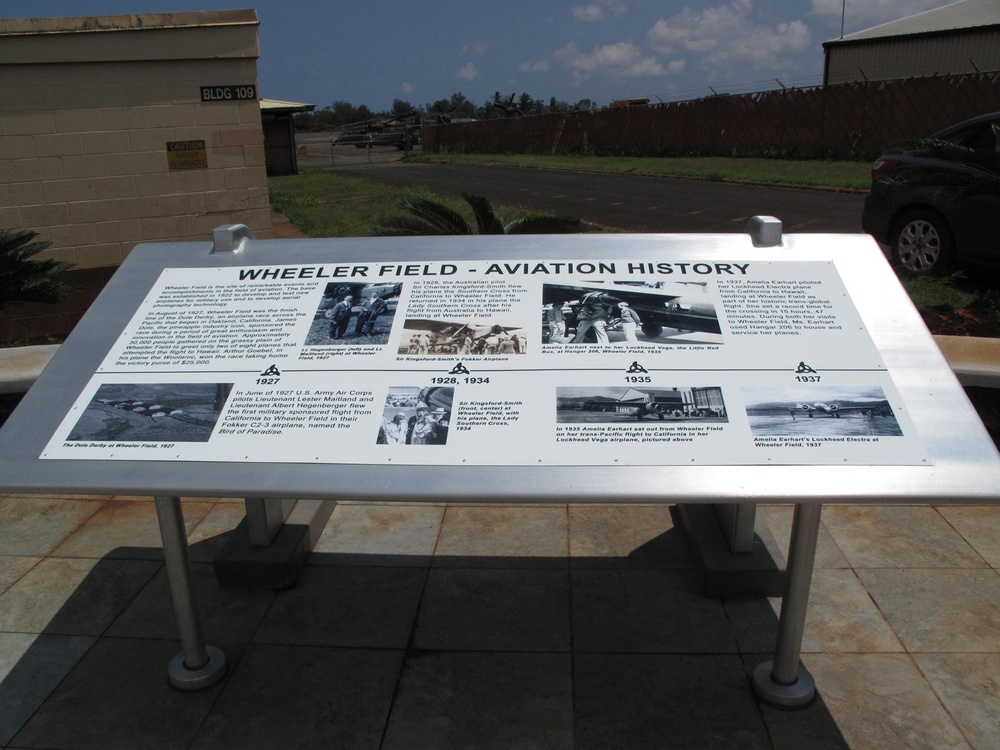This horizontal rectangular image appears to depict an outdoor museum display at dusk, just as the sky transitions to a dark grayish-blue hue. The scene features a silver plaque holding what looks like a page of text and images, suggesting it is explaining historical content. The top of the plaque prominently displays the title "Wheeler Field - Aviation History" in bold black letters, followed by several lines of smaller black print. The display includes seven unarranged black-and-white photographs that likely chronicle the field's development and significant events.

The plaque, reflective and possibly placed on a table with cylindrical and rectangular legs, stands in an open area with visible surroundings. To the right side of the image, a car can be seen on a road next to a fence, surrounded by grassy patches and trees. Several buildings are also visible, illuminated by the remaining daylight, indicating the photograph was taken with some natural light still remaining. This setting hints at a historical site dedicated to aviation history, particularly of Wheeler Field, with mentions of key dates like its opening in 1927 and subsequent events up to 1934. Despite details on the plaque being too small to read clearly in the image, aircraft activities such as takeoffs or landings are faintly visible, elevating the historical narrative of the celebrated field.